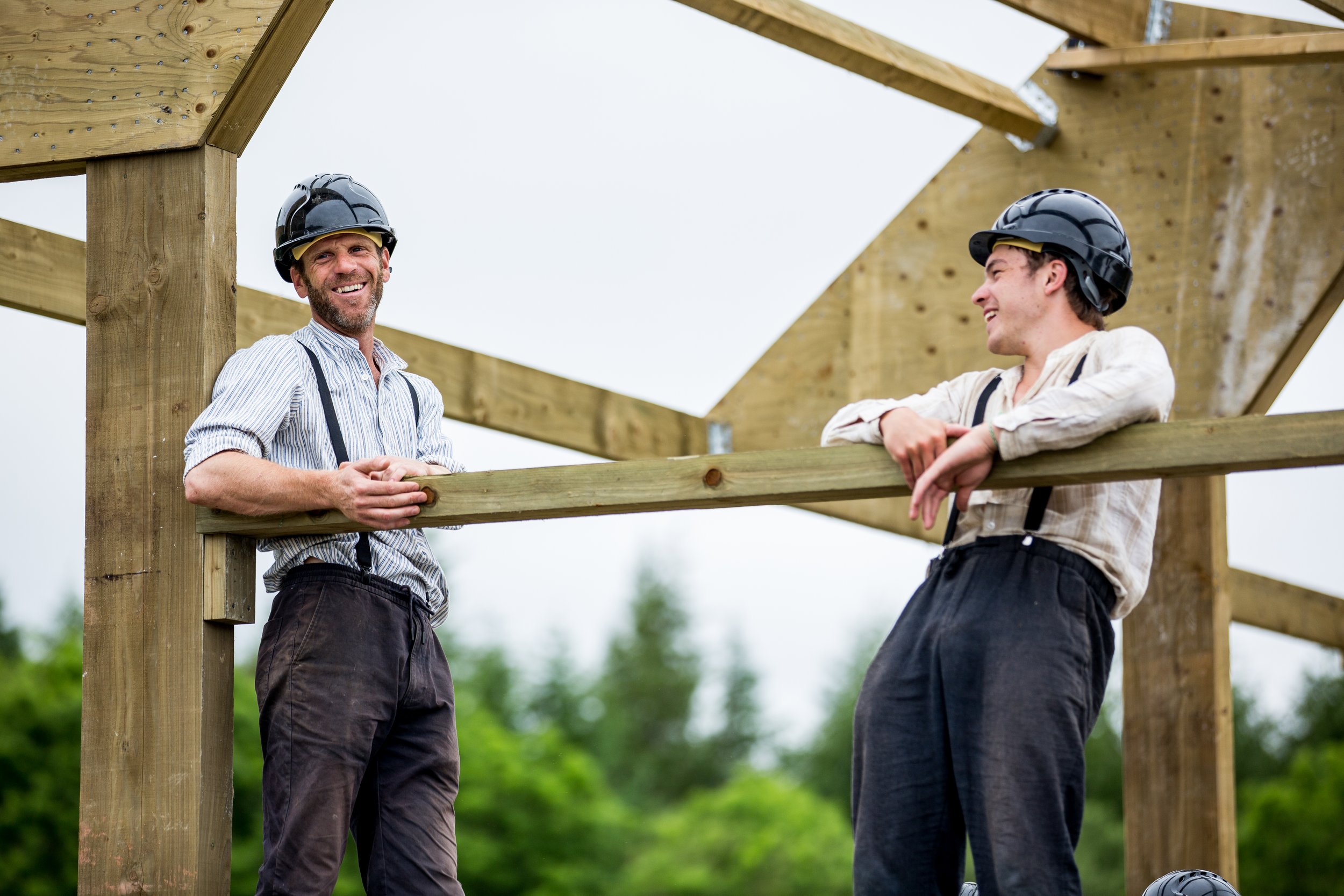This photograph captures two construction workers, possibly Amish or Mennonite, engaged in building a new structure, likely a barn or house. The men, clad in dark pants, suspenders, and button-front shirts, are perched on an elevated work platform. Both are wearing black construction helmets with yellow forehead bands but no chin straps. The man on the left, who appears middle-aged with grizzled facial hair, smiles warmly at his younger companion, who seems to be a teenager or in his early twenties. This younger man gazes directly at the camera, also smiling. Both men exude happiness and camaraderie as they lean against a horizontal wooden beam, hands casually hooked over it. Their feet are not visible, as the photo is cropped below the knees. The background features a dense wooded area with a mix of rounded deciduous trees and tall evergreen trees, all under a bright white sky. The wooden structure they are working on is clearly in the early stages of construction, with fresh, unweathered lumber forming the skeletal framework, devoid of siding or roofing. A third construction helmet is faintly visible at the bottom right corner, hinting at the presence of another worker.